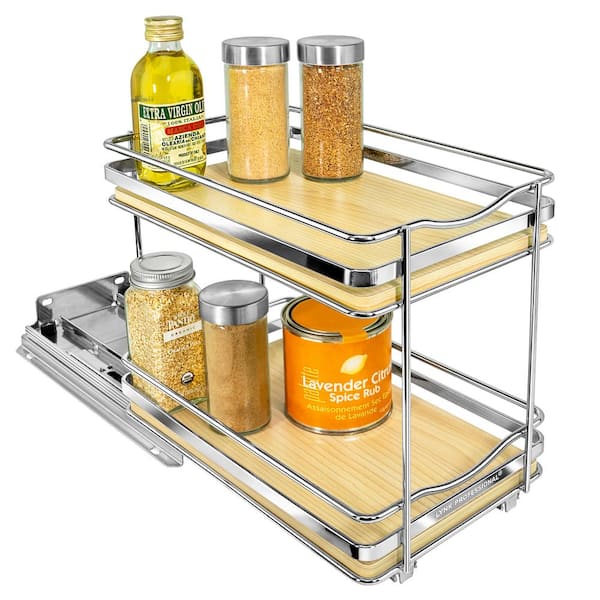The image is a highly detailed, color photograph in a square format showcasing a stainless steel, two-tiered slide-out shelf organizer designed for kitchen cabinets. The organizer features a sleek chrome finish with a mounting bracket on the back for securing it to the underside of a cabinet, allowing it to be easily pulled out and pushed back for convenient access. Each of the two shelves has light wood-colored bases and is fitted with chrome guardrails that prevent items from falling off. The structure is reinforced with four vertical chrome supports — two at the front and two at the back. The top shelf holds a bottle of extra-virgin olive oil in the back left corner, flanked by two jars of spices to its right. The bottom shelf is arranged with several more jars of spices, including an orange can of spice. The composition is minimalistic and emphasizes the practicality and design of the product against a clean, white background, exemplifying photographic representational realism in product photography.